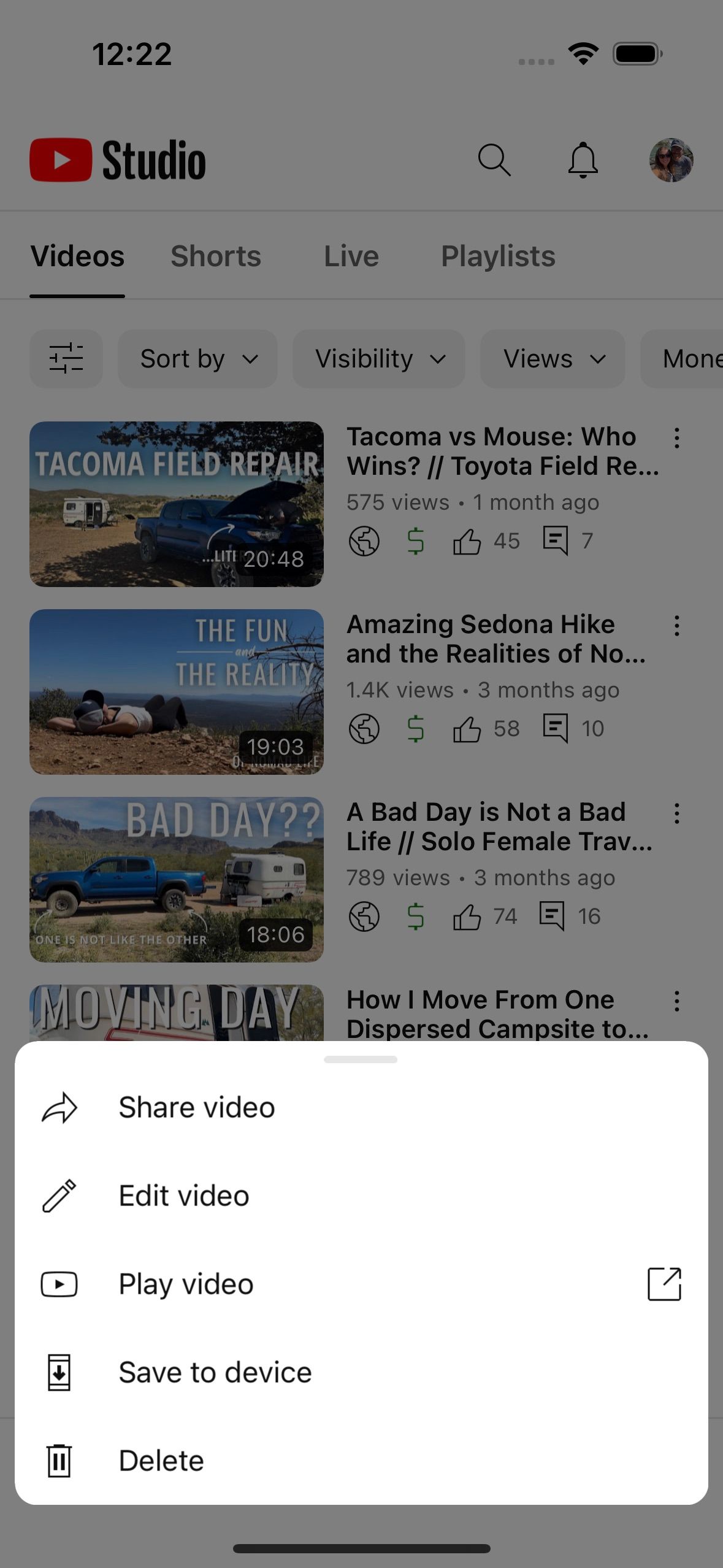A screenshot displays a YouTube-like interface at the time 12:22. Key elements include a studio icon, a magnifying glass (search function), a notification bell, and a profile picture. Tabs available are "Videos" (underlined, indicating the current view), "Shorts," "Live," and "Playlists." 

A sorting option labeled "Sort by: Visibility, Views" is also present. The video list comprises:

1. **Title:** "Tacoma vs. V.S. Muse: Who Wins? Toyota Field RE..."
   - **Views:** 575
   - **Posted:** 1 month ago
   - **Icons:** Globe, Dollar Sign
   - **Engagement:** 45 likes, 7 comments

2. **Title:** "Amazing Students, Amazing Sedona Hike, and the Realities of..."
   - **Views:** 1.4K
   - **Posted:** 3 months ago
   - **Icons:** Globe, Dollar Sign
   - **Engagement:** 58 likes, 10 comments

3. **Title:** "Has a Bad Day, It's Not a Bad Life: Solo Female Trav..."
   - **Views:** 789
   - **Posted:** 3 months ago
   - **Icons:** Globe, Dollar Sign
   - **Engagement:** 74 likes, 16 comments